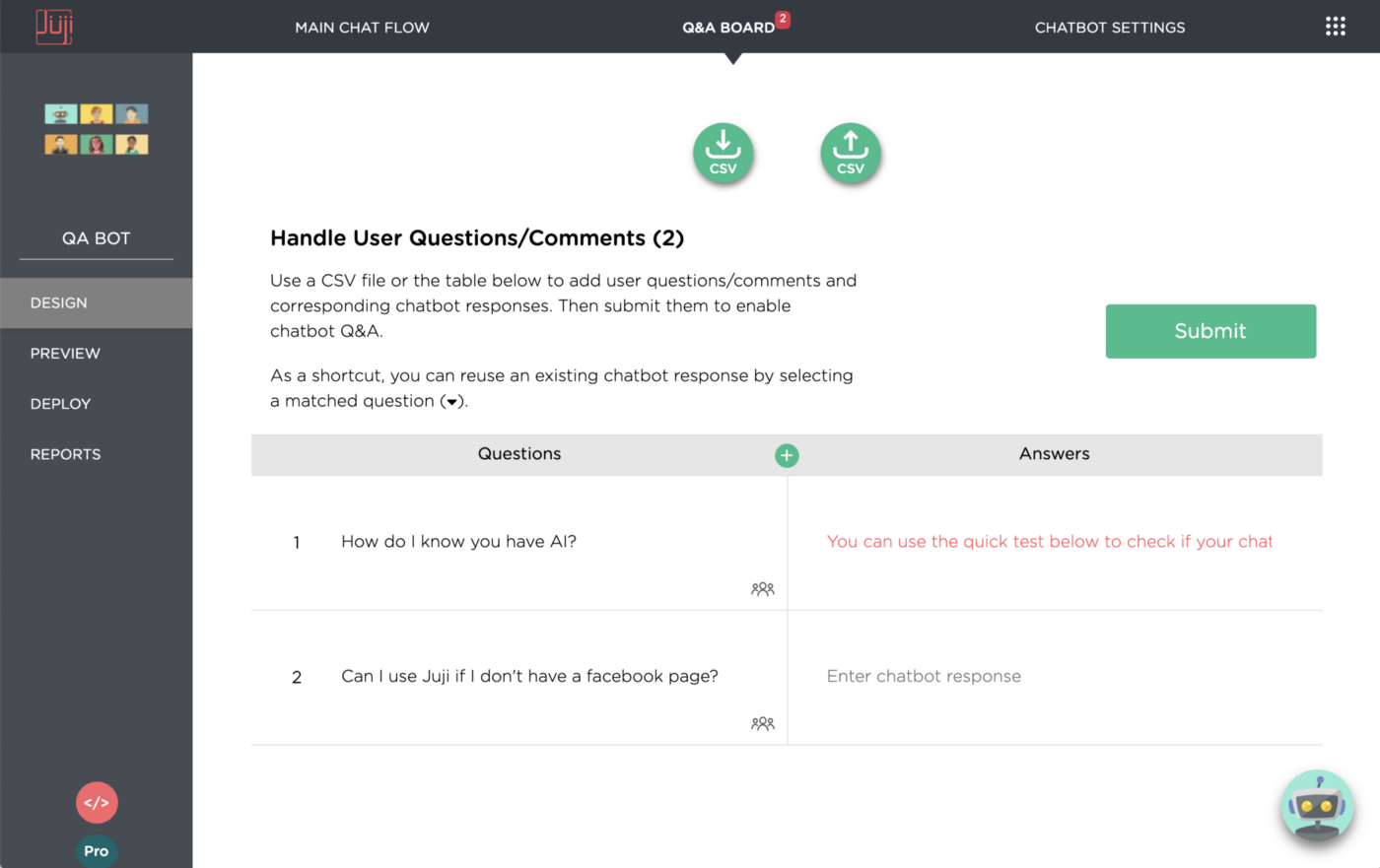This image is a landscape-format, color screenshot of a website called "Juji." The website's logo "Juji" is prominently displayed at the top in red text, with a capital 'J' and lowercase 'uji,' where the 'u' features an umlaut, giving it a unique, slightly Japanese aesthetic. The logo is set against a black banner background, which also contains white text navigation options, including "Main Chat Flow," "Q&A Board," and "Chatbot Settings." The "Q&A Board" section notably has a small indicator showing the number "2," suggesting there are two questions present.

In the center of the page, instructions read: "Handle user questions/comments. Use the CSV file or the table below to add user questions/comments and the corresponding chatbot responses, then submit them to enable chatbot Q&A." Below this, specific questions and their responses are listed. The first question displayed is "How do I know you have AI?" with a partially visible response stating "You can use the quick test below to check if your chat," and the rest is cut off. The second question shown is "Can I use Juji if I don't have a Facebook page?" with a blank space indicating there's currently no response entered for this query.